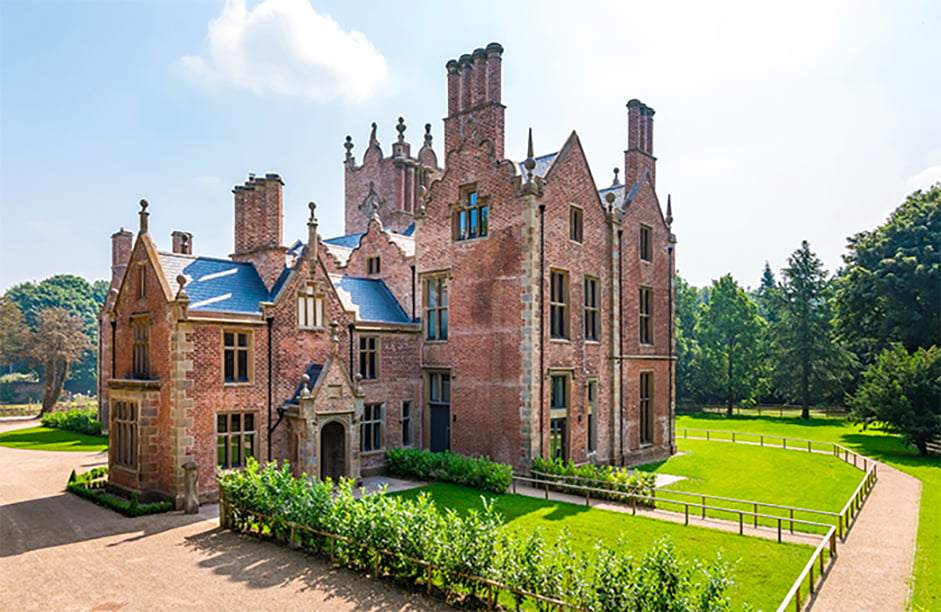The image captures an expansive, older brick building that strongly resembles a mansion or small palace with a castle-like design. Constructed primarily from red, burnt pink brick, it features multiple peaks and numerous chimneys, at least seven in total with over ten chimney flutes. The roof is covered in gray shingles and adorned with elaborate turrets and pillars, giving it an almost institutional or religious architectural style. Lining the building are many large, tall windows, and it has a prominent arched doorway. 

The structure appears to be well-preserved, suggesting little to no additions since its original construction. Surrounding the building is a well-manicured green lawn bordered by short wooden post fencing along the pathways, and some minimal shrubbery without notable flowers. In the back, a dense mixture of evergreen and deciduous trees, full of leaves indicating summertime, frames the mansion against a partly cloudy sky with patches of blue. The overall setting hints at a grand residence, suitable for a large family, with an air of historical significance and quiet elegance.